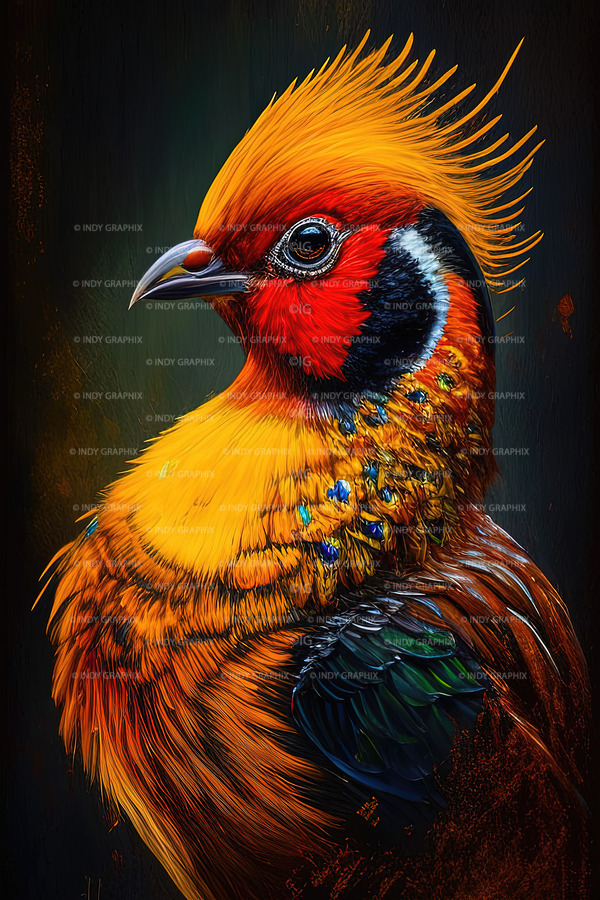The digitally-created image showcases a unique bird with a mixture of vivid colors and intricate details against a dark green background, which fades to a lighter shade in the center. Overlaid on the image is translucent white text reading "Indie Graphics" to denote copyright. This imagined bird features an orange crown with feather projections, adorned with blue and green glittery hearts, adding an unrealistic touch. It has a distinctive face marked with red around its eyes and black behind that. The bird's beak is small and gray, and its chin and neck area are yellow, leading down to an orangish-brown body with a mix of green and black on the wings. Additional details include brown eyes, blue spots on the neck, and black and white markings, creating a visually striking composition.